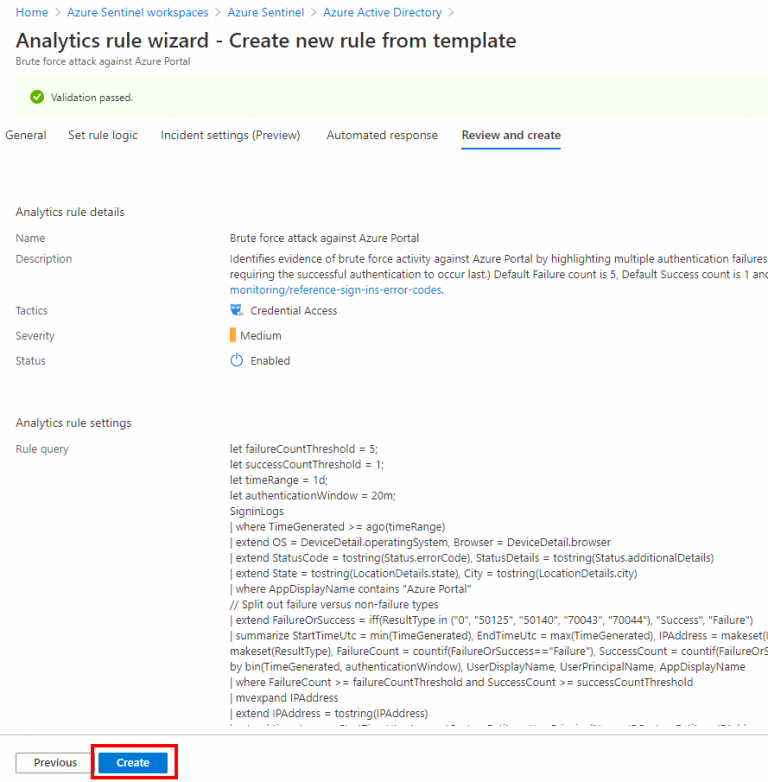This image depicts a screenshot of a web page interface. In the top left-hand corner, there are four horizontally arranged categories highlighted in blue font. These categories are labeled, from left to right: "Home," "Azure Sentinel Workplaces," "Azure Sentinel," and "Azure Active Directory." Beneath these categories is a prominent title in bold text that reads: "Analytics Rule Wizard - Create New Rule from Template." Just below this title, there is an indication that the verification has passed, marked by a white check within a green circle. The main body of the screenshot provides detailed descriptions including fields such as "Name," "Tactics," "Severity," "Status," and "Rule Settings." At the bottom left-hand corner, there are two option buttons: "Previous" on the left and "Create" on the right. The "Create" button is highlighted with a red outline and is blue in color, whereas the "Previous" button is white.